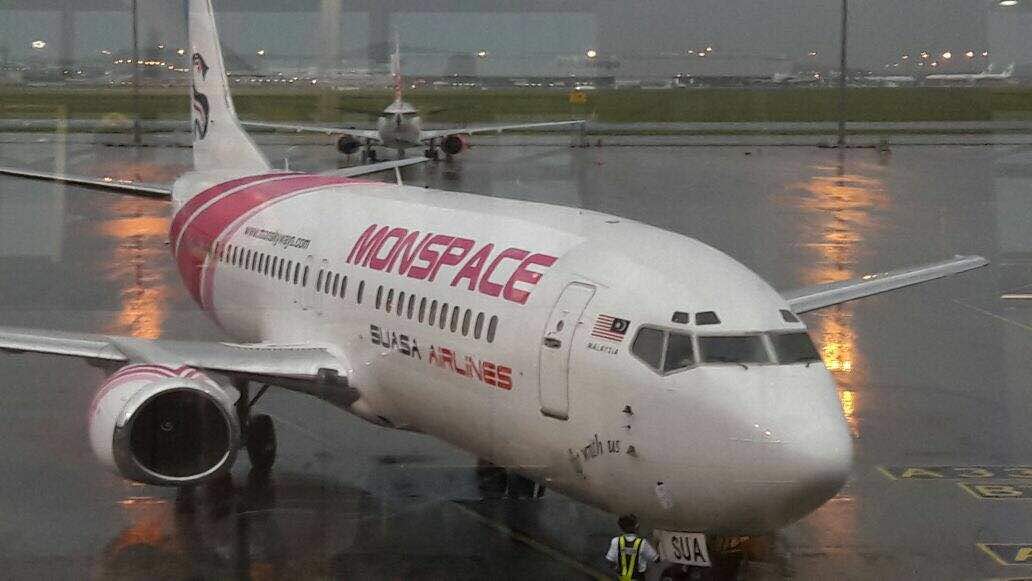This is a horizontally aligned photographic image captured at an airport during the evening, with the wet surface of the runway reflecting orange lights. The focal point is a white jet airplane prominently featuring the red lettering "M-O-N-S-P-A-C-E" along its side, signifying its association with Suasa Airlines, marked also by the "S-U-A-S-A" lettering underneath the nose. The airplane carries a red, white, and blue Malaysian flag with the word "Malaysia" inscribed on it, and a silver band accentuates the jet engine. Additionally, there is a man in a yellow and black safety vest nearing the airplane's front end. In the background, another jet and buildings with lights on can be seen under the gray sky. The tarmac, appearing wet and dark gray, extends into the distance, featuring a grassy field and buildings beyond. The tail of the airplane showcases an 'S' and a red band, while the web address "www.suasaairline.com" is vaguely visible on the jet in the background.